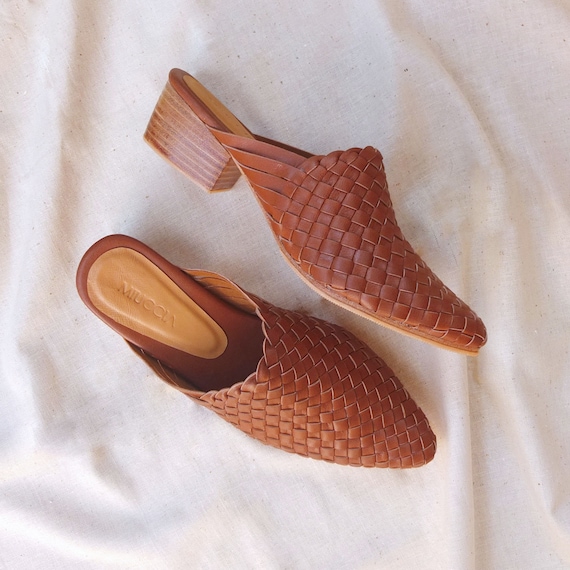This photograph, taken from a top-down perspective, showcases a pair of women's sandals placed on a white cloth background. One sandal is positioned straight, while the other is tilted sideways, revealing both a direct and a side view. The sandals are crafted from brown leather, featuring a crisscross pattern on the front half which is covered, and an open back half. A design in light brown is embellished on the back portion, with the brand name "Miyucha" imprinted on it. The cushioned heel area is in a yellow buttery shade. The sandals have chunky, brown-colored heels, notable for their layered wood texture. Overall, the sandals appear new and unworn.